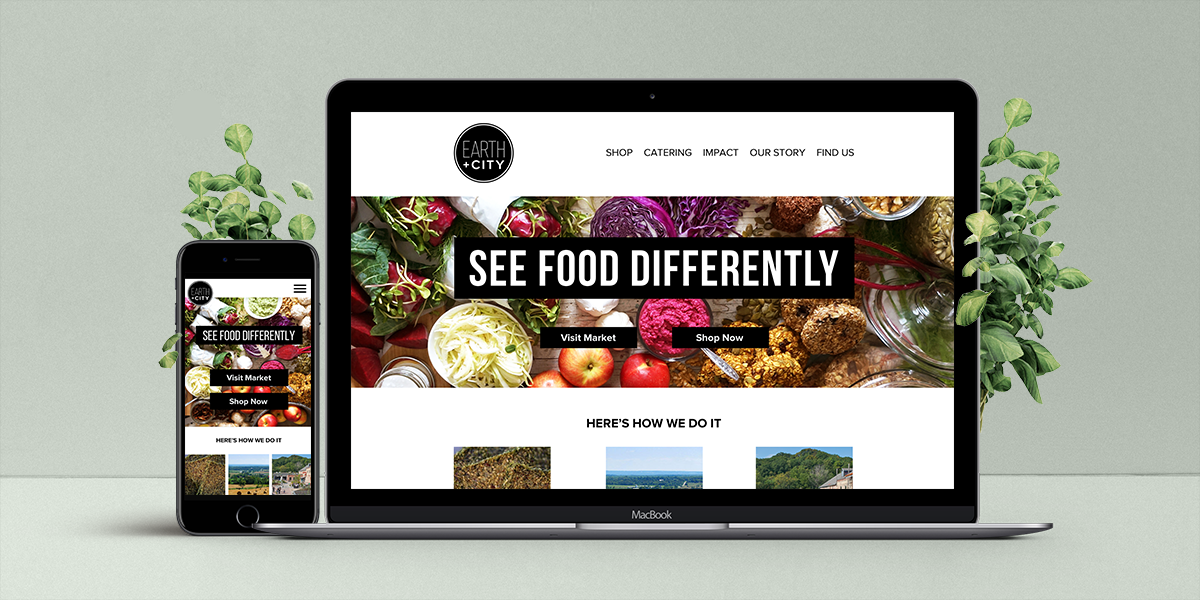The image displays a laptop screen positioned at the top, showcasing a website header with the options "Shop," "Catering," "Impact," "Our Story," and "Find Us." The text "Earth City: Here's How We Do It" is prominently featured. Next to the laptop, a smartphone displays the exact same webpage. The background is predominantly white, with the exception of a central section filled with vibrant and appetizing pictures of various dishes. The overall white background enhances the focus on the showcased food imagery, emphasizing the theme "I See Food Differently."